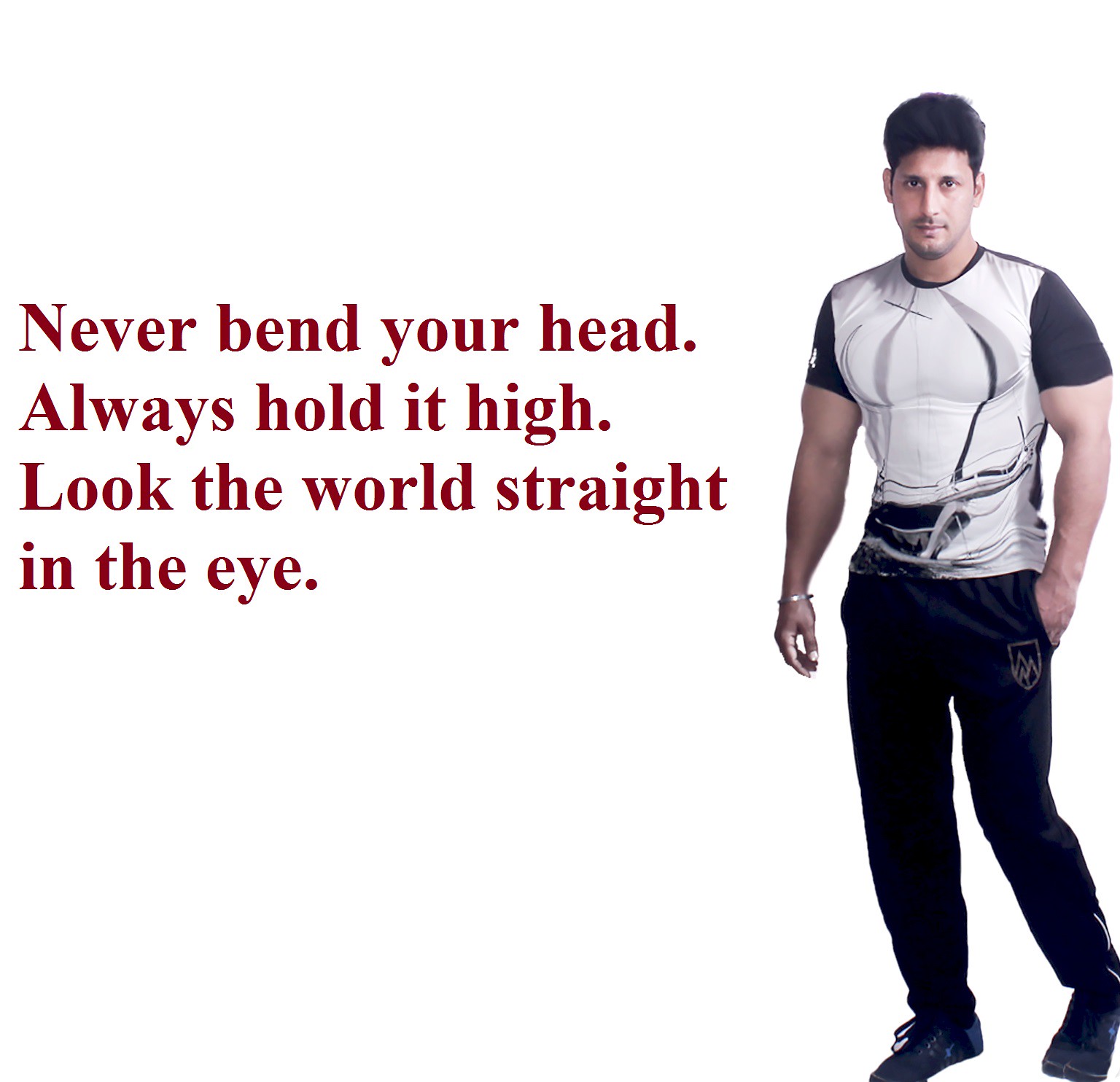In this image, a muscular, brown-skinned man with short black hair stands confidently to the right, his serious gaze directed straight at the camera, embodying the spirit of the adjacent text. He wears a snug black and white t-shirt, which highlights his fit physique, along with black workout pants and black and blue sneakers. His left hand rests in his pocket, and a silver bracelet adorns his right wrist. Details, including his slight stubble and tall hair, add to his composed and steadfast appearance. The white background is stark and uncluttered, focusing attention entirely on the subject and the motivational quote in dark maroon-red text to the left, which reads: "Never bend your head, always hold it high. Look the world straight in the eye." This phrase aptly complements the man's poised and determined posture.